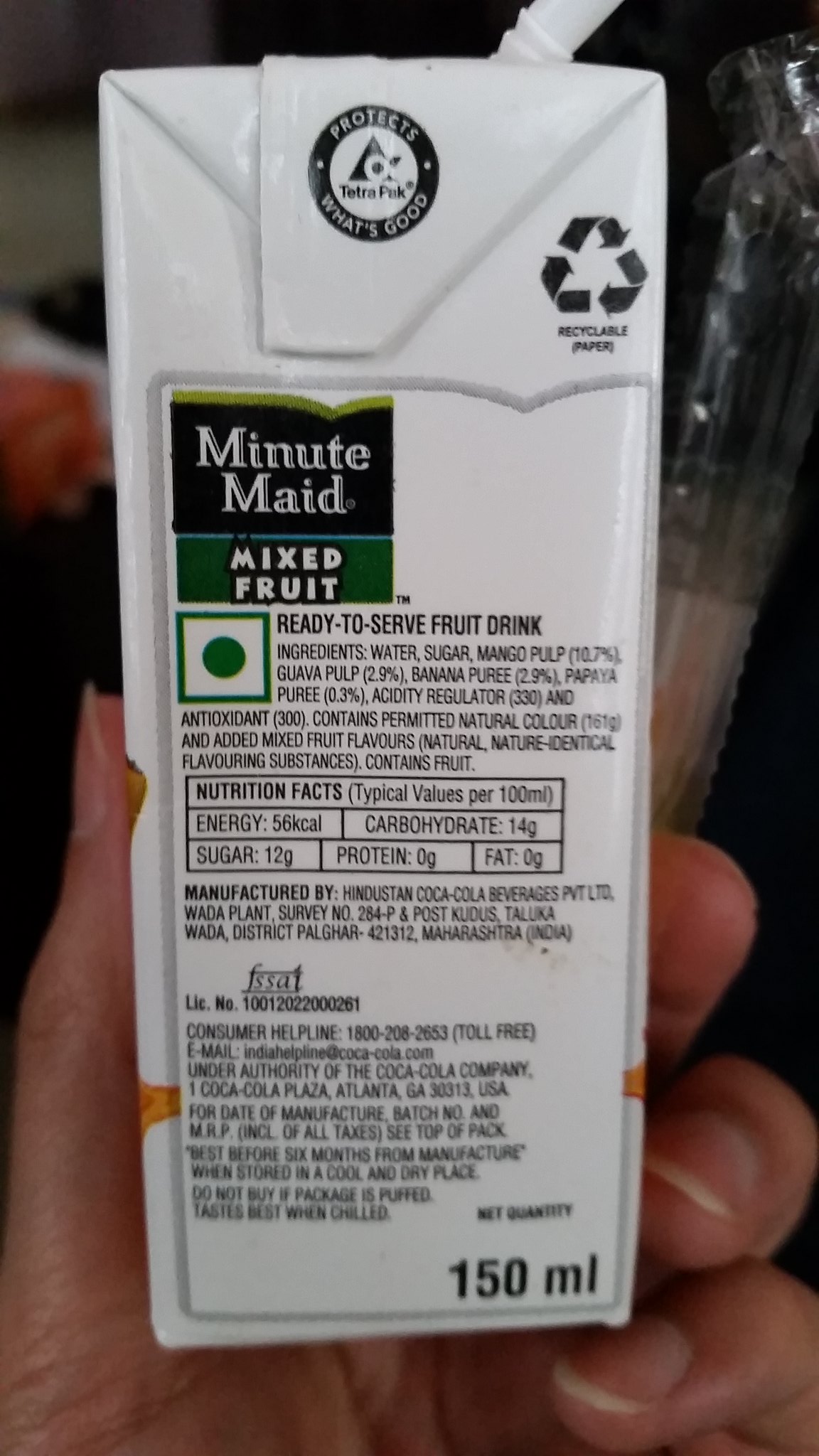A photograph captures a person holding a small, single-serve white juice box with their hand partially visible, showing fingers and thumb. The carton is a Minute Maid Mixed Fruit juice box, prominently labeled with "Minute Maid" in black with white text, followed by "Mixed Fruit" set on a black and green background with a thin turquoise line between them. The side of the box lists the ingredients in black text, starting with water, sugar, mango pulp (10.7%), guava pulp (2.9%), banana puree (2.9%), and papaya puree (0.3%). Additional contents include acidity regulator 330, antioxidant 300, permitted natural color, natural, nature, and whole growing substances, and added mixed fruit flavors. At the top, it reads "Ready to Serve Fruit Drink." Also visible is a black recyclable icon at the top right. The net quantity, 150 milliliters, is marked at the bottom, and a plastic straw encased in a wrapper emerges from the top of the box. The photograph includes a slightly blurred background, emphasizing the focus on the juice box's detailed information.